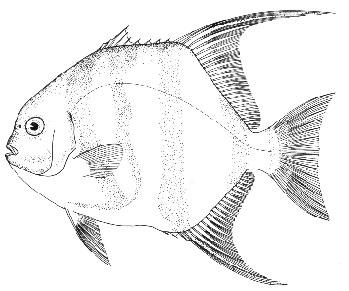This black and white hand-drawn sketch depicts a flat, rounded fish pointing to the left, with its mouth slightly open, taking up almost the entire image. The fish's body, possibly resembling a flounder or sunfish, is broad and tall, showcasing its distinct dorsal and bottom fins. Its large, round eye with a black pupil is prominently featured on the left side, just above a small crest-like fin on its forehead. The fish exhibits a striking pattern with light-colored vertical stripes extending down its body and through its various fins, giving it a unique texture. From the side view, it appears slim, with notable details including two side fins—one smaller fin towards the front and a larger one near the tail. The tail itself is short, rounded, and curves slightly back into the body, completing the fish's streamlined yet chonky appearance.